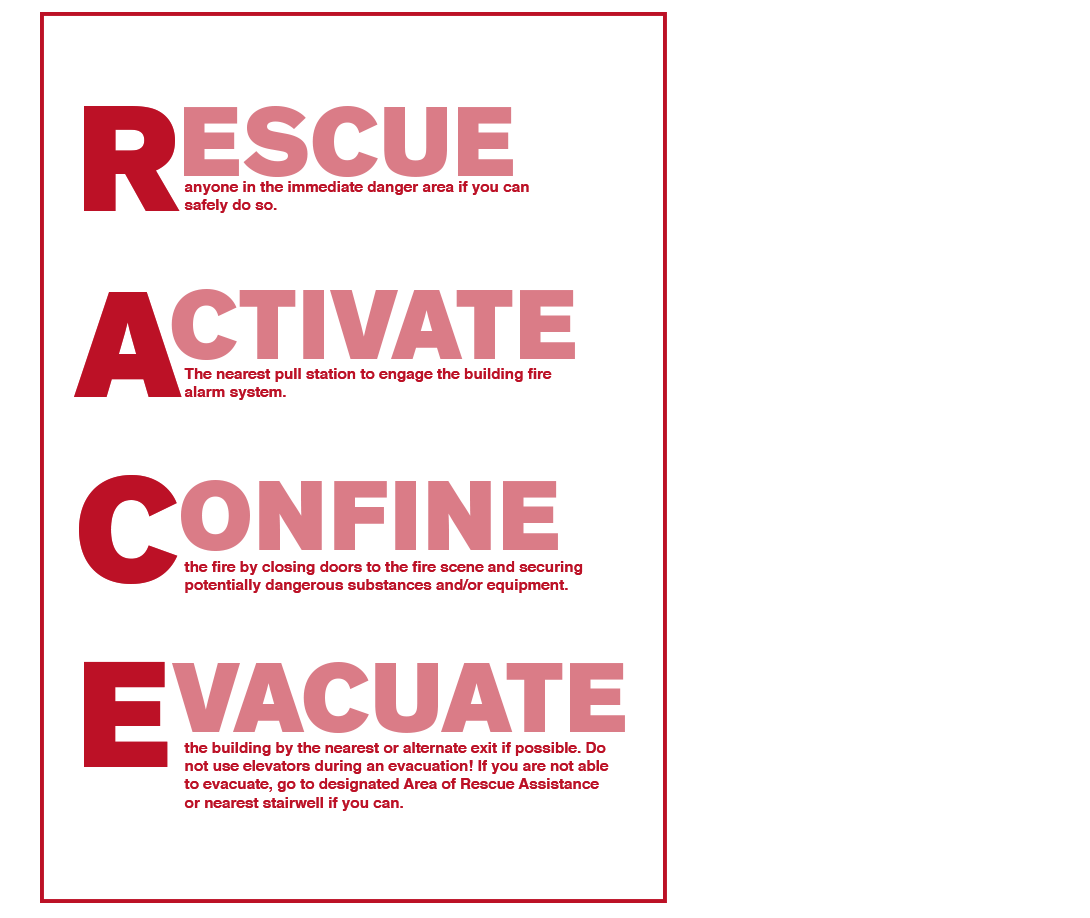This image depicts a detailed and essential instructional poster designed for fire response teams, including first responders such as firefighters and police. The poster, bordered by a thin red outline on a white background, prominently features the acronym "R-A-C-E" vertically in bold red capital letters. Each letter in the acronym stands for a crucial step in fire emergency protocol: 

- **R for Rescue**: Rescue anyone in the immediate danger area if you can do so safely.
- **A for Activate**: Activate the nearest pull station to trigger the building’s fire alarm system.
- **C for Confine**: Confine the fire by closing doors to the fire scene and securing potentially dangerous substances or equipment to starve the fire of oxygen.
- **E for Evacuate**: Evacuate the building using the nearest or alternate exit if possible, and avoid using elevators. If evacuation isn't possible, proceed to the nearest stairwell or designated area of rescue assistance.

The poster's design emphasizes the importance of these steps by using darker and bolder red letters for the acronym, making it clear and easily readable both vertically and horizontally. This visual aid serves as a quick reference guide during fire emergencies, reinforcing critical actions to protect life and property.